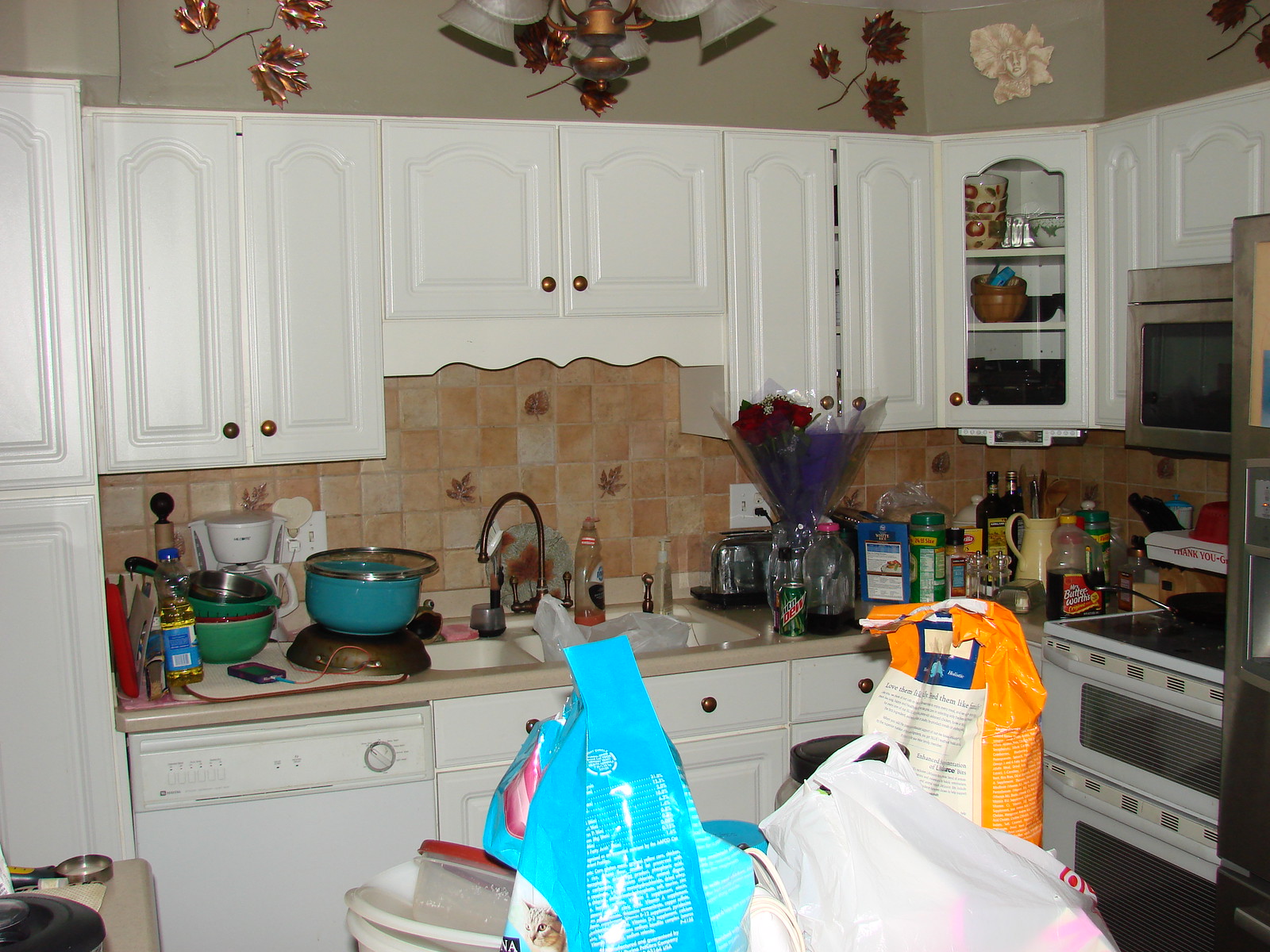In this detailed photograph, the upper section showcases a brownish top of the walls adorned with intricate bronze leaf designs on the left, which transition into a bronze branch with leaves in the adjacent sections. In the middle of the composition, an elegant light fixture with glass components casts an intricate shadow. The fixture appears to have silver, white, and possibly hints of gold accents, with a partially obscure face and surrounding design.

Beneath this, the kitchen features pristine white cabinets and drawers, each accented with copper handles. The backsplash is a mixture of brown and light grey tiles, perfectly matching the cabinetry. On the far right corner, an open shelving unit adjacent to a silver microwave adds functionality. Below a beige countertop, which includes dual white sinks with grey taps, sits a white dishwasher.

A black-top stove with white, elongated handles, and a silver fridge can be seen to the right of the sinks. The countertop hosts an assortment of items including an orange bag with a white label, a blue bag, and a clear plastic bag in the center. To the right of the sink stands a toaster and a white electrical socket. In front of the socket is a green Mountain Dew can with a red label. A plant with red rose-like flowers is also visible, along with various bottles and kitchenware.

On the countertop is a blue pot with a glass lid, perched atop an upside-down grey frying pan. Beside these, a phone is seen charging near a white coffee machine with glass components in the background.